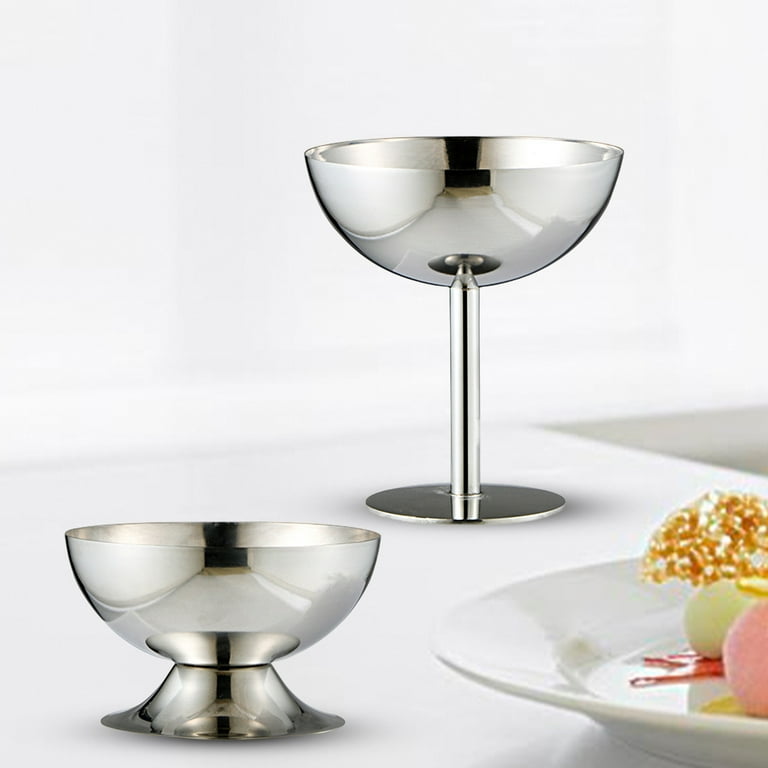In the image, we see a variety of sophisticated tableware and some ornate delicacies presented on a white surface against a white wall background. On the upper right, there's a sleek silver goblet with a thin stem and a shiny, reflective surface. To its left is a smaller silver bowl, sharing the same metallic finish but with a wider base suitable for holding nuts or small snacks. In the bottom right corner, partially cut off, is a shallow white plate adorned with intricate dessert arrangements. These desserts appear to be ice cream balls, with a mix of light green and red tones, crowned with delicate golden crunchies that resemble an umbrella-like design. The meticulous presentation evokes a sense of luxury and culinary artistry.